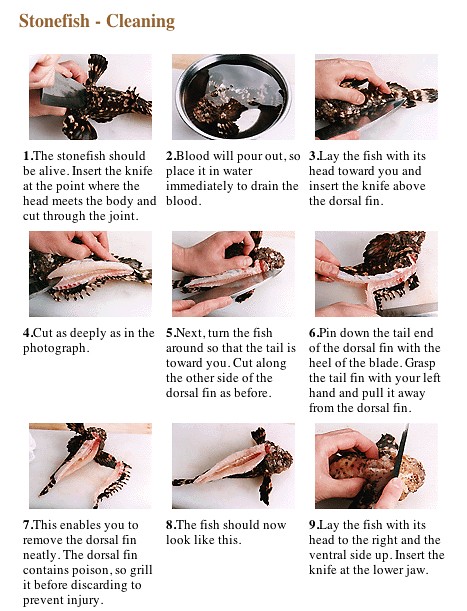This color image titled "Stonefish Cleaning" features a detailed, step-by-step photographic guide to cleaning a stonefish, arranged in a 3x3 grid format totaling nine photos. The sequence progresses from the top row (steps 1-3), through the middle row (steps 4-6), to the bottom row (steps 7-9).

1. The stonefish should be alive. Insert the knife at the point where the head meets the body and cut through the joint.
2. Blood will pour out, so place the fish in water immediately to drain the blood.
3. Lay the fish with its head toward you and insert the knife above the dorsal fin.
4. Cut deeply as shown in the photograph.
5. Turn the fish around so that the tail is toward you and cut along the other side of the dorsal fin.
6. Pin down the tail end of the dorsal fin with the heel of the blade, grasp the tail fin with your left hand, and pull it away.
7. This enables you to remove the dorsal fin neatly. Be cautious; the dorsal fin contains poison, so grill it before discarding to prevent injury.
8. The fish should now appear as shown in the corresponding photo.
9. Lay the fish with its head to the right and the ventral side up, inserting the knife at the lower jaw.

The stonefish itself exhibits colors such as brown, pink, and some black, while the accompanying bowl is silver. The instructional text is in black. The setting is simple and functional, aimed at effectively conveying the cleaning process through both text and images.